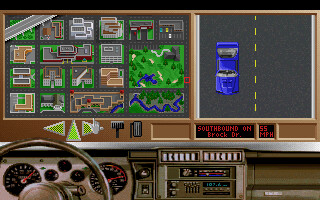This rectangular screenshot from a simple-looking driving video game is divided into three main sections. The top half of the image is further split into two distinct areas. On the left, an overhead map displays a fictional landscape featuring buildings, parks, and rivers, depicting the in-game environment. On the right, an overhead shot of a blue car is seen navigating a two-lane road marked by yellow serrated lines. The car occupies the left lane with its front facing the bottom of the image.

The bottom third of the screenshot reveals an interior view of the car's dashboard, showcasing an old-style steering wheel in a light brownish-greyish hue. Behind the steering wheel are five black dials: two larger ones on the outside and three smaller dials arranged in a triangular configuration. Below these is an old-fashioned radio with a digital display showing green digits, flanked by a blue and red line, which suggests climate control settings. Above the radio, air conditioning vents are visible.

Occupying the space just above the dashboard view, there are images of the car's brake and accelerator pedals, indicating the player's control inputs. The image annotation "southbound on Brock Drive at 55mph" in red font provides additional context about the car's current status in the game. This detailed composition captures the essence of a straightforward driving game, featuring both in-game navigation and the car's dashboard interface.